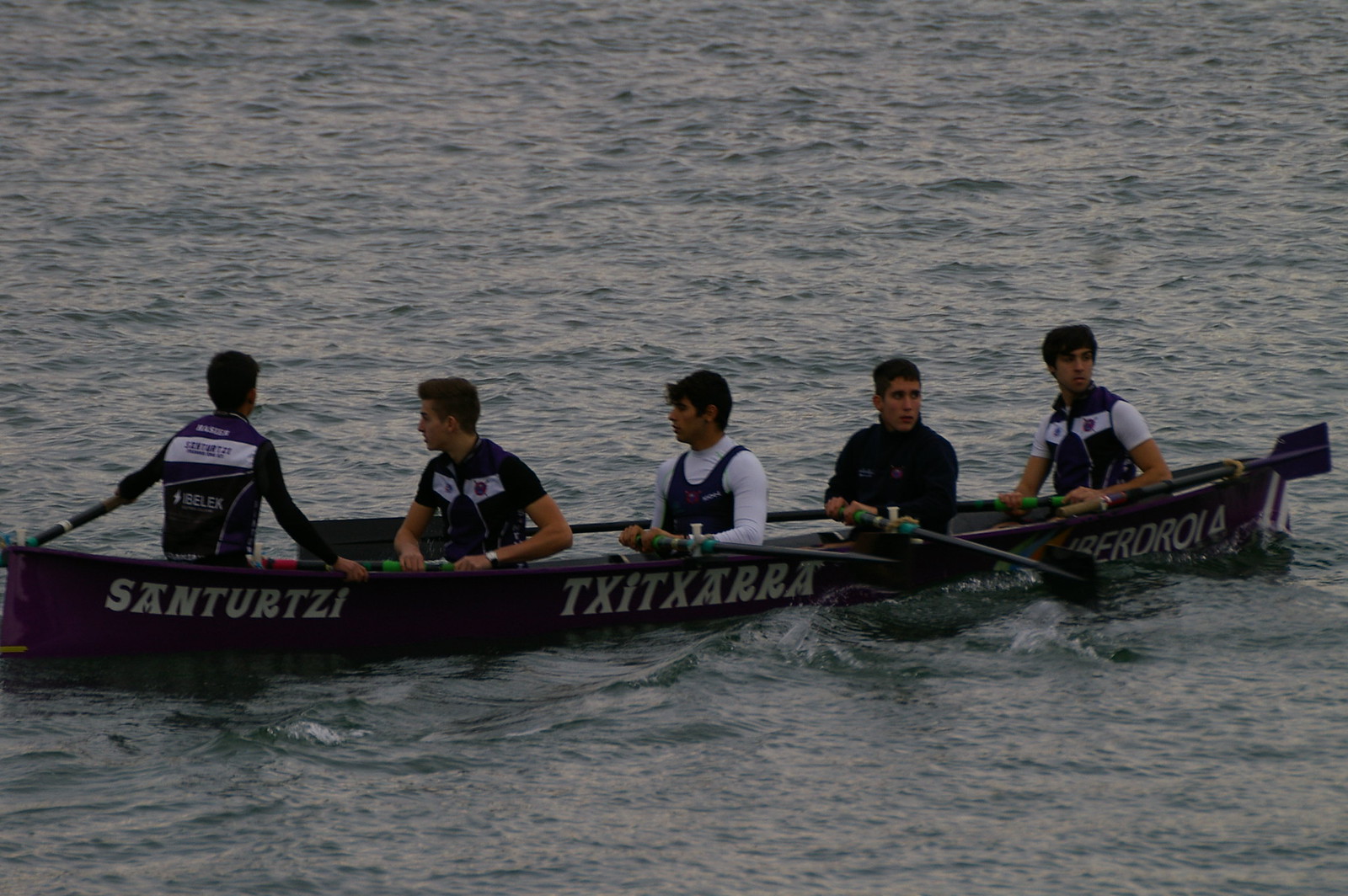In the image, five men are seated in a long, dark-colored canoe, approximately 30 feet in length, rowing across the water in what appears to be dusk. The boat, surrounded by blue-tinted water, bears white inscriptions in a foreign language: "S-A-N-T-U-R-T-Z-I" on the left, "T-X-I-T-X-A-R-R-A" in the middle, and "R-E-R-O-R-O-I" on the right. All five rowers are equipped with black paddles and are dressed for potential water immersion, wearing jackets and varied types of clothing for potential safety. The man at the far left, facing away from the camera, dons a black outfit with a prominent white stripe on his back, possibly showcasing his name. Directly to his right, the rowers have contrasting attires: one in all-black long sleeves, another in a white long sleeve shirt with a black tank top over it, and another sporting a white shirt with a black and white vest. The far-right rower is identifiable by his short white sleeve shirt paired with a protective jacket featuring white rectangles, possibly flag-like patches. They all appear to be synchronized in their rowing, highlighting the structured coordination essential for the sport.